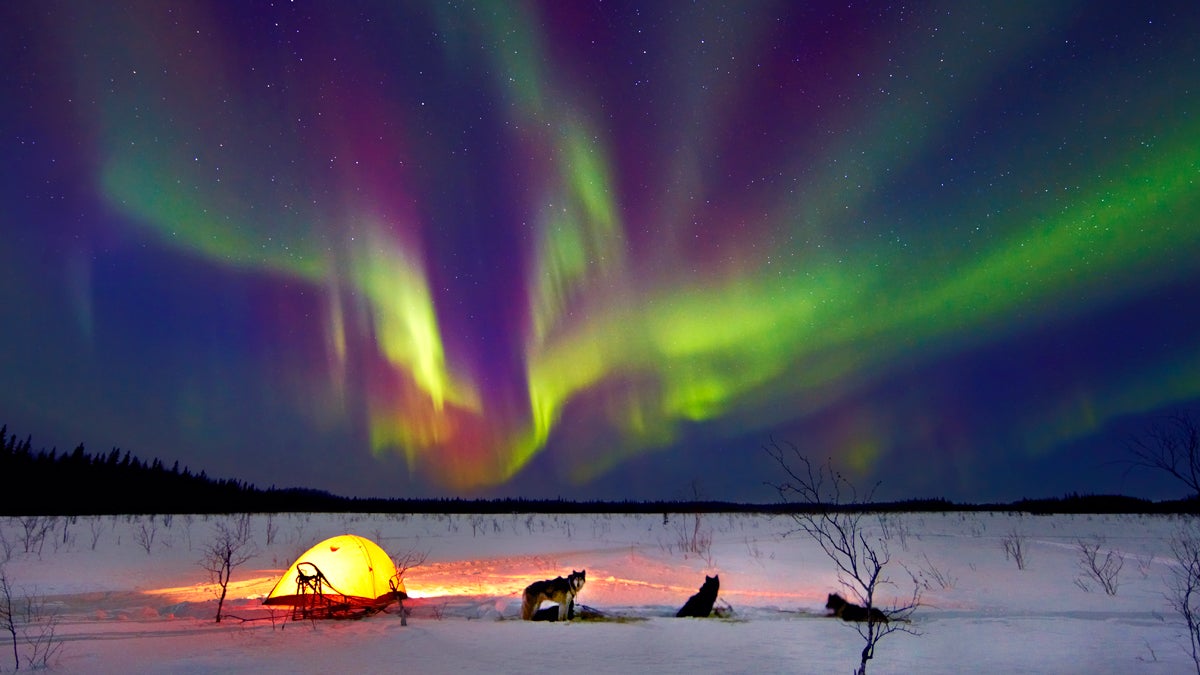This stunning photograph captures a mesmerizing winter scene with snow blanketing the ground and a vibrant aurora borealis dominating the night sky. The sky is a spectacular display of bright green and purple hues, with accents of yellow and hints of orange along the horizon. In the foreground, a sled team of six Siberian huskies, some standing and some laying down, is positioned near a glowing yellow-orange two-man tent, lit from within by a lantern. Scattered small pines and twig-like trees punctuate the snowy plains, leading to hills covered in dense pine trees in the background. The brilliant aurora, reflected in the snow and enhancing the scene, captivates both the viewer and the sled dogs, seemingly gazing at the northern lights. Every detail, from the star-studded sky to the trail marked by the sled, is vividly clear, contributing to the overall beauty and luminosity of the photograph.